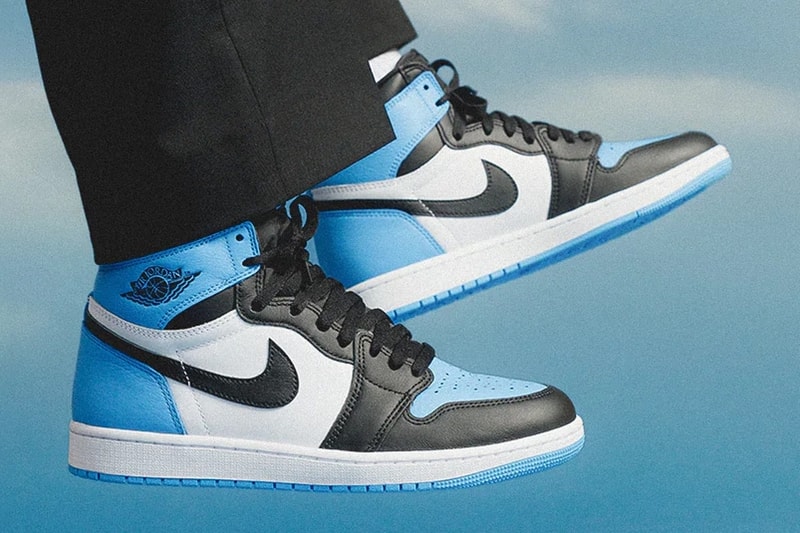This advertisement showcases a close-up of a person's feet wearing a pair of high-top Nike Air Jordan shoes against a vivid blue background that resembles a cloudy sky. The shoes, primarily composed of black, white, and blue leather, are accentuated by black laces and feature a distinctive black Nike swoosh that starts in the middle of the shoe and wraps around the back. The back of the shoes and the textured soles are a sky blue, harmonizing with the backdrop. Above the intricately detailed basketball emblem with ornate wings is the 'Air Jordan' script, suggestive of a classic, potentially vintage, design. The person is wearing black slacks, causing the stylish shoes to stand out prominently in the image.